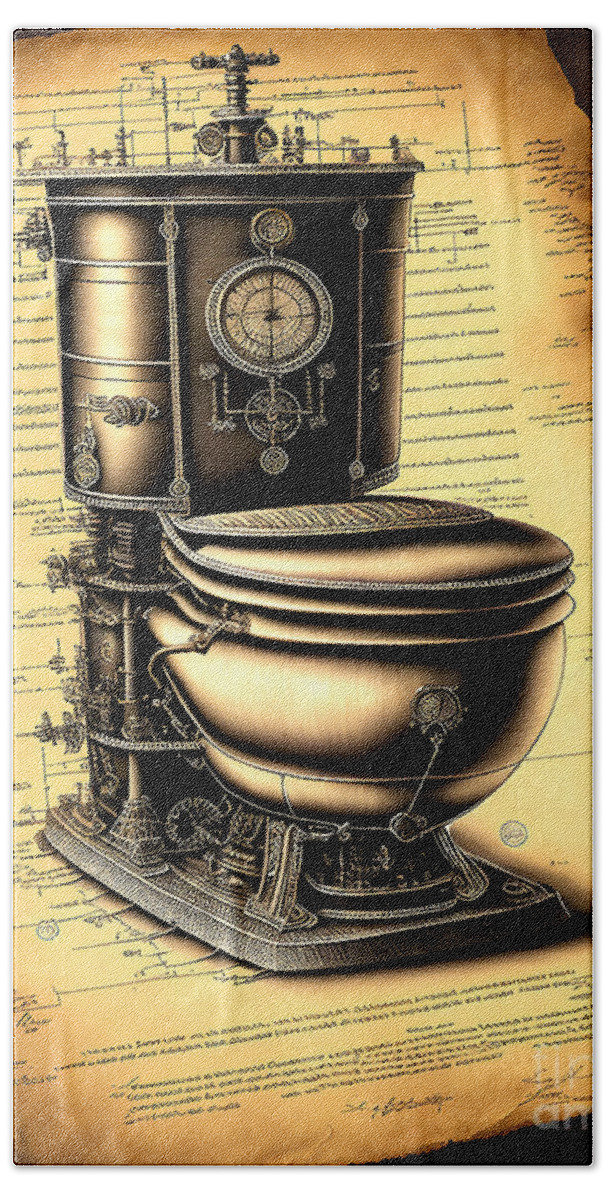The image depicts a vintage, bronze-colored toilet with an intricate and ornate design. Positioned in front of an aged, yellowish-gold paper covered with unreadable handwriting, this antique piece stands out with its detailed craftsmanship. The toilet features a turning handle at the top and a golden seat, complemented by various gauges and possibly a compass-like dial. The toilet is mounted on a dark gray, elaborately decorated base, with additional metal elements and wires extending from it. The extensive old paper behind the toilet might include explanatory notes or design schematics related to this peculiar artifact.